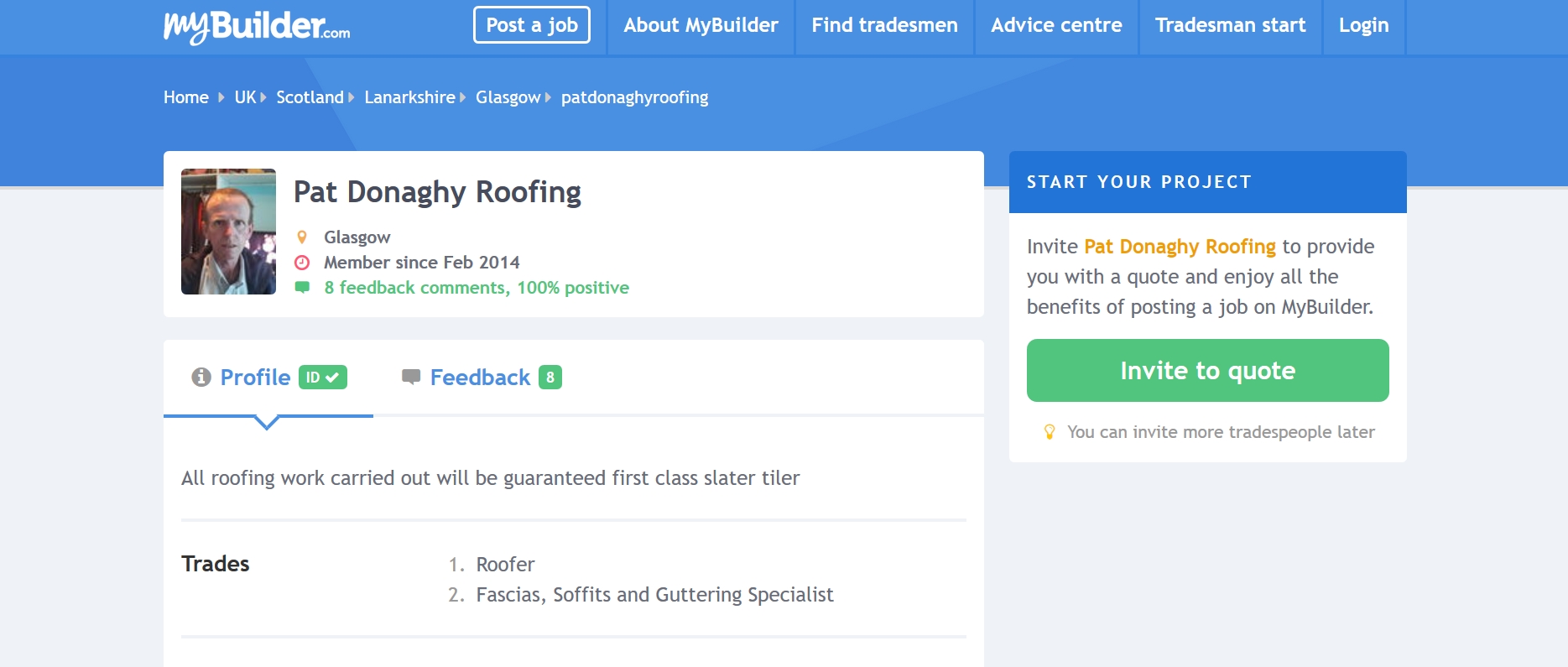This screenshot captures a webpage from MyBuilder.com, set against a blue background. The top navigation bar prominently features buttons for "Post a Job," "About MyBuilder," "Find Tradesmen," "Advice Centre," "Tradesmen Start," and "Login." Breadcrumb navigation below traces the user's path: Home > UK > Scotland > Lancashire > Glasgow > Pat Donahue Roofing.

Currently, the page focuses on "Pat Donahue Roofing," showcasing a profile image of a man with brown hair, dressed in a white shirt and black jacket. The profile details reveal that the business is based in Glasgow and has been a member of MyBuilder since February 2014. Impressively, they have received eight feedback comments, all of which are 100% positive.

The profile elaborates on their expertise, stating that all roofing work is guaranteed to be first class. The trades listed include roofer, slater, tiler, and guttering specialist. A call-to-action message on the side encourages users to start their project by inviting Pat Donahue Roofing to quote. A green "Invite to Quote" button is available, with a note indicating that additional tradespeople can be invited later.

The page's design primarily features a white background with black text, while the top section has a lighter blue background with white buttons.